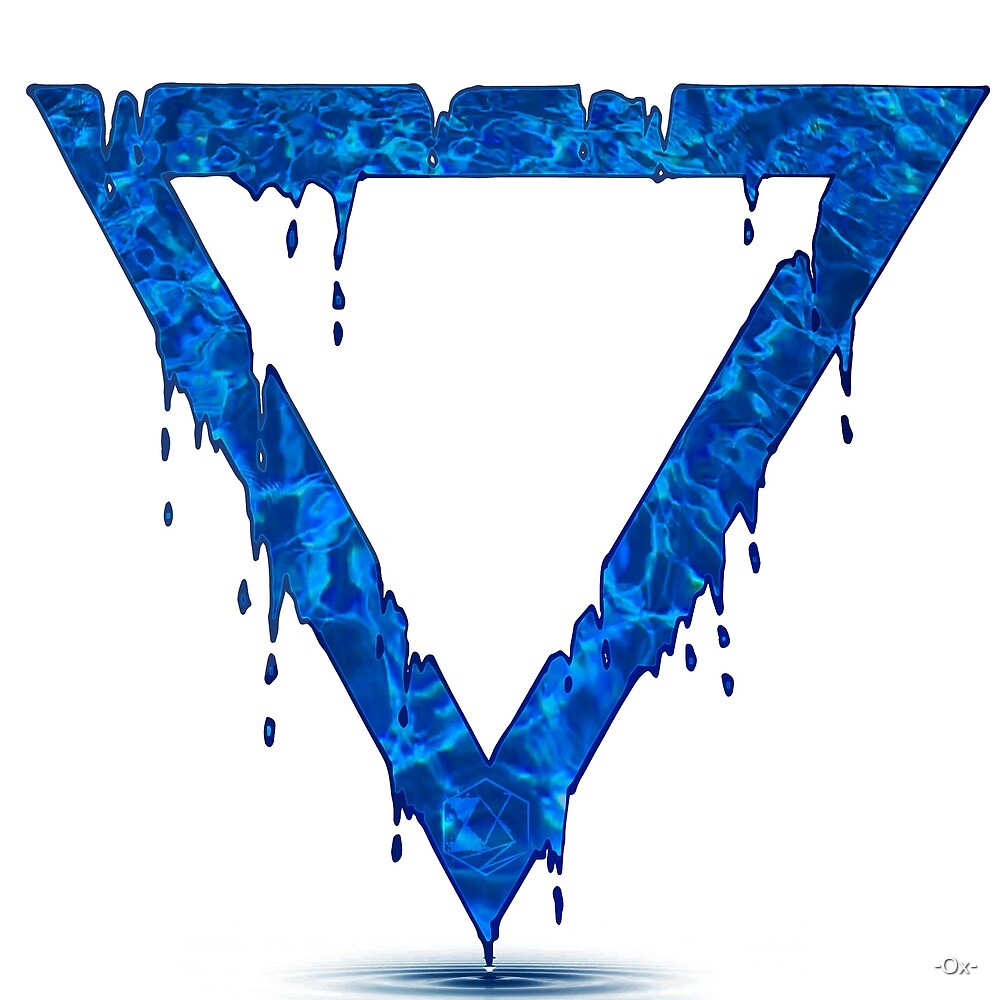This is an image of an upside-down triangle with a striking graphic design. The triangle features a thick, irregular blue outline, which varies in shades from dark to light blue and even bluish-gray highlights. Along its edges, the blue appears to be dripping, resembling wet paint or melting icicles, creating an impression that the triangle is slowly disintegrating or freshly painted. Intriguingly, parts of the blue material seem to be breaking away, further adding to the melting effect. The center of the triangle is hollow, exposing a white background that contrasts sharply with the vivid blue border.

At the very tip of the triangle's point at the bottom, there is a small, noticeable hexagonal shape with an X and a Z inside of it, contributing to a logo-like appearance. This tip seems to be dipping into a small blue puddle, creating ripples that enhance the image's fluid, dynamic quality. The entire scene is suggestive of water reflections, much like looking into a rippling pool. This combination of dripping, melting effects, varied blue shades, and reflective water elements gives the image a rich, textured, and almost surreal aesthetic.